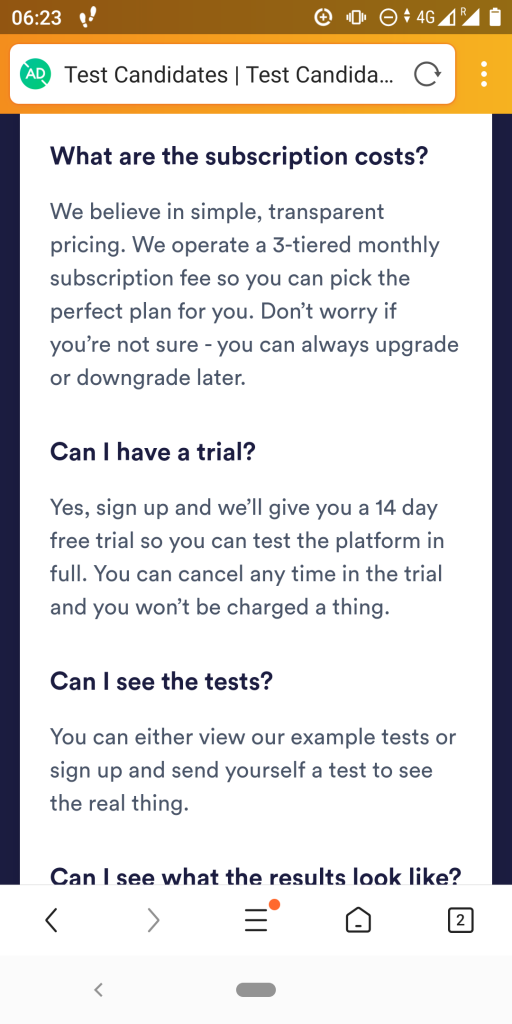This image depicts a mobile screenshot captured on a smartphone, shown in a vertical layout. 

In the top left corner, the time reads 6:23, while the right corner displays a 4G signal indicator and a mostly charged battery icon. Below this, an orange status bar is followed by a white search bar with the text "test candidates" written twice, accompanied by a refresh icon to the right. To the left of the search bar, there is a green circle containing the letters "AD."

Below the search bar is a white vertical rectangle with thin navy blue stripes running up on either side of the text. This section contains black text detailing subscription costs and trial information: 

"What are the subscription costs? We believe in simple, transparent pricing. We operate a three-tiered monthly subscription fee so you can pick the perfect plan for you. Don't worry if you're not sure, you can always upgrade or downgrade later.

Can I have a trial? Yes. Sign up and we'll give you a 14-day free trial so you can test the platform in full. You can cancel any time in the trial and you won't be charged a thing.

Can I see the tests? You can either view our example tests or sign up and send yourself a test to see the real thing."

At the bottom of the screen, a navigation bar features a backward arrow, a forward arrow, a menu with three horizontal dots, a home icon, and a square icon with the number "2" inside it.